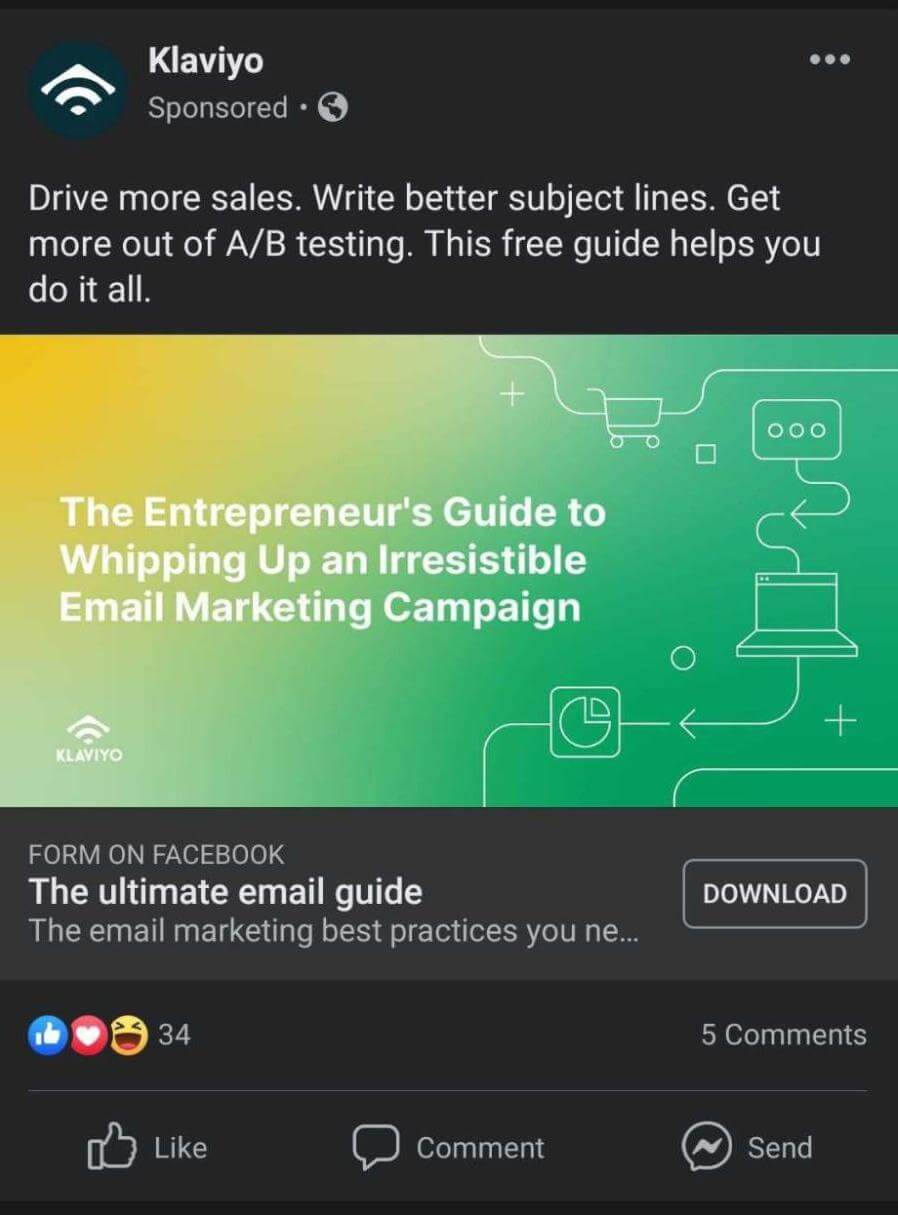This detailed description captures the elements prominently present in the sponsored Facebook ad by Klaviyo. You can use this as a refined and comprehensive caption for the image:

---

A Facebook ad screenshot from Klaviyo, marked as sponsored with an earth icon, encourages users to engage with a free comprehensive guide aimed at enhancing their email marketing strategies. The promotional blurb invites users to drive more sales, craft better subject lines, and optimize A/B testing. The featured image showcases a yellow-to-green ombre background, adorned with minimalistic, white-line graphics including a shopping cart, a message bubble, a computer, a small pie chart, and arrows connecting all elements. The text overlaid on the image, in prominent white font, reads "The Entrepreneur's Guide to Whipping Up an Irresistible Email Marketing Campaign," with Klaviyo's logo in the bottom left corner. Beneath the image, a continuation of the blurb reads "form on Facebook, the ultimate email guide, the email marketing best practices you ne..." trailing off with a download button. Interaction options such as like, comment, and send are available at the bottom of the post.

---